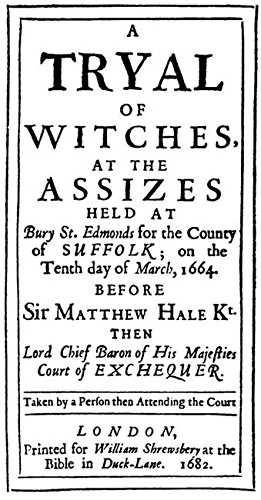This black-and-white image is a rectangular poster bordered by two thin black lines, creating a high-contrast framed effect around the text. This vintage document, printed in 1682 by William Shrewsbury at the Bible in Duck Lane, serves as a detailed record of a historic witch trial held on March 10, 1664. The trial took place at the Assizes in Bury St. Edmunds for the County of Suffolk, overseen by Sir Matthew Hale, then the Lord Chief Baron of His Majesty's Court of Exchequer. The document’s text features varied font sizes, with the word "trial" notably spelled in an old-fashioned manner as "T-R-Y-A-L." The caption indicates that this was taken by an individual attending the court, reflecting the formal language and typography of the era.